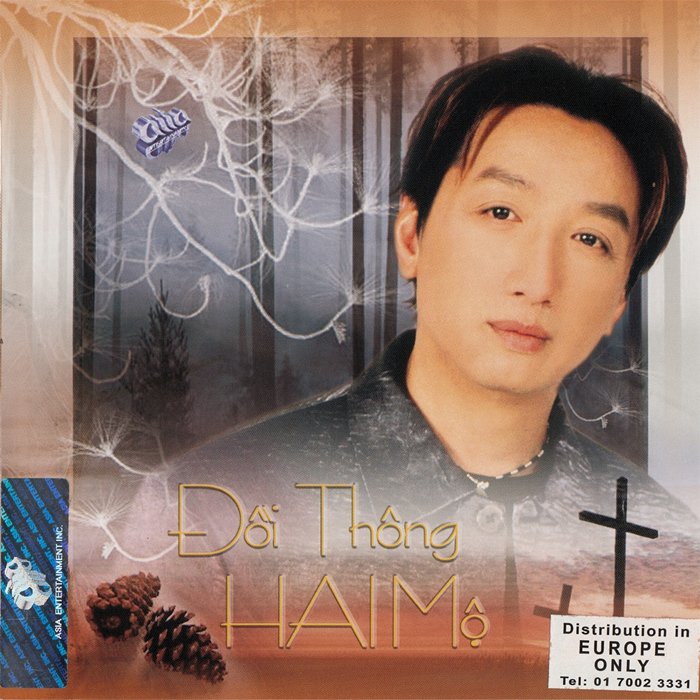The image features a close-up of a young, attractive Asian man from the shoulders up. He has short, dark hair that is parted, visible ears, and pink lips. He is wearing a black shirt with white accents and a beaded necklace. The background is a misty forest with added white drawings of branches and daisy flowers. In the lower corners, there are two pine cones in the left and two crosses in the right. Additionally, there's a yellow square labeled "Asian Entertainment Incorporated" and a notice that says, "Doin Thong Hamon, Distribution in Europe Only, Telephone: 01-7002-3331." This appears to be a poster or album cover, featuring the man against an ethereal, superimposed background of trees on a gray, cloudy day.